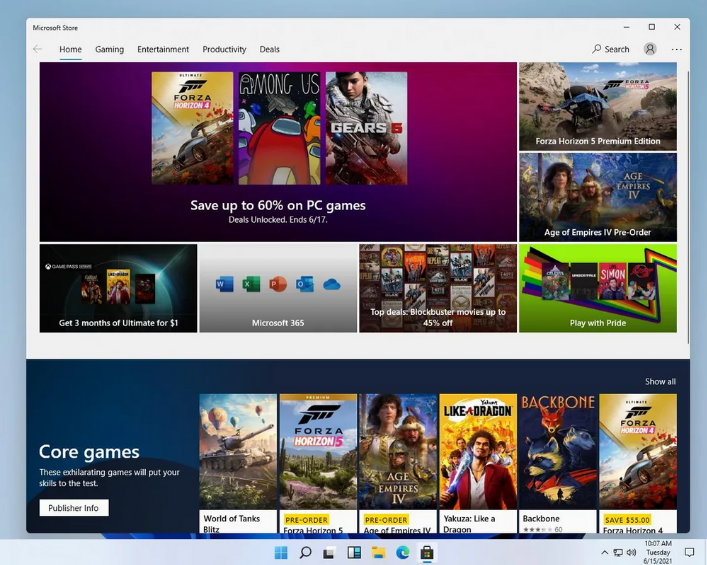A screenshot of a Microsoft Store web page captures a comprehensive layout despite missing the top section. On the left, the page is titled "Microsoft Store," and on the right, there are options to minimize, maximize, or close the window. The main navigation bar at the bottom includes options for "Home," "Gaming," "Entertainment," "Productivity," and "Deals," with a search function and user avatar options located on the extreme right.

The significant visual elements include a prominent top rectangle banner with a gradient purplish hue that showcases three games—Forza, Among Us, and Gears—and an enticing offer boasting up to 60% off on PC games, with the promotion ending on June 17. Adjacent to this banner, a vertical arrangement of images features Forza Horizon, Age of Empires, and a "Play with Pride" section, indicating a themed event.

Lower on the page, a section titled "Core Games" introduces a selection of challenging games designed to test players' skills, including titles like World of Tanks, Forza Horizon S, Age of Empires 4, Like a Dragon Backbone, and Forza 4. Users have the option to click for more information or view all these exhilarating game offers.